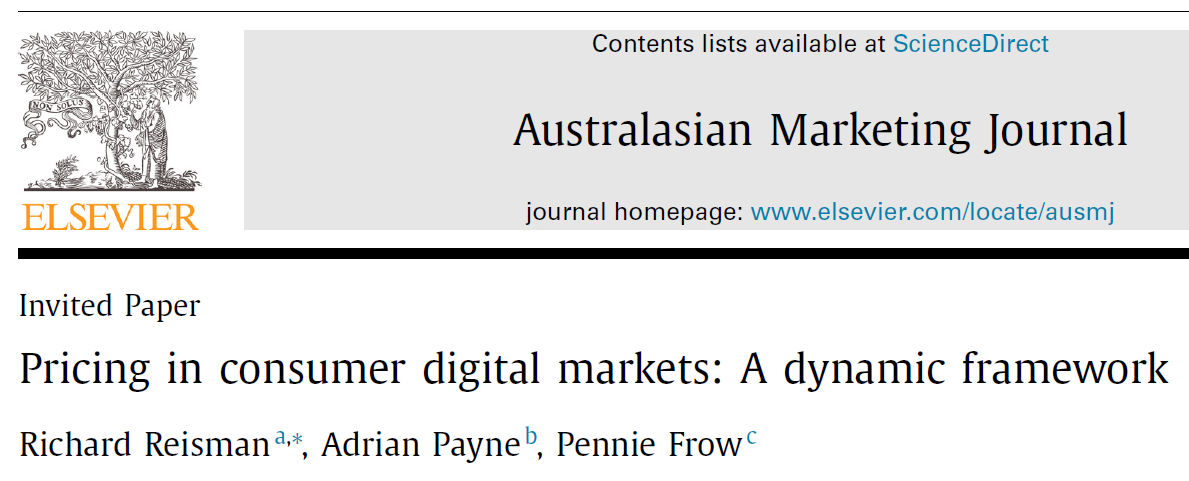This image is a screenshot of a professional magazine or journal page, presented with a minimalistic design on a white background. At the top of the page, there is a small rectangular banner. On the left side of this banner, an intricate black-and-white illustration of a tree, replete with numerous leaves and branches, adds a touch of detailed artistry. Adjacent to the tree illustration, the name "Elsevier" is prominently displayed in bold orange letters, signifying the publisher's identity.

Right next to this visual display, a gray rectangle contains essential navigation information. At the top of this gray section, a concise line of text reads, "Contents List Available at ScienceDirect," with the term "ScienceDirect" highlighted in blue. Dominating the center of the banner, large bold black letters declare the title "Australasian Marketing Journal." Beneath this major title, the words "Journal Homepage" are printed in a smaller black font. Directly following, the URL "www.elsevier.com/locate/AUSMJ" is displayed in blue, providing a direct link to the journal's online presence.

A distinct dark black line separates the banner from the content below. Following this line, the label "Invited Paper" is printed in smaller letters. The main title of the featured paper, "Pricing and Consumer Digital Markets: A Dynamic Framework," is presented in larger prominent letters. The authors of the paper—Richard Rosman, Adrian Payne, and Penny Froude—are listed underneath, indicating their contribution to the scholarly work.